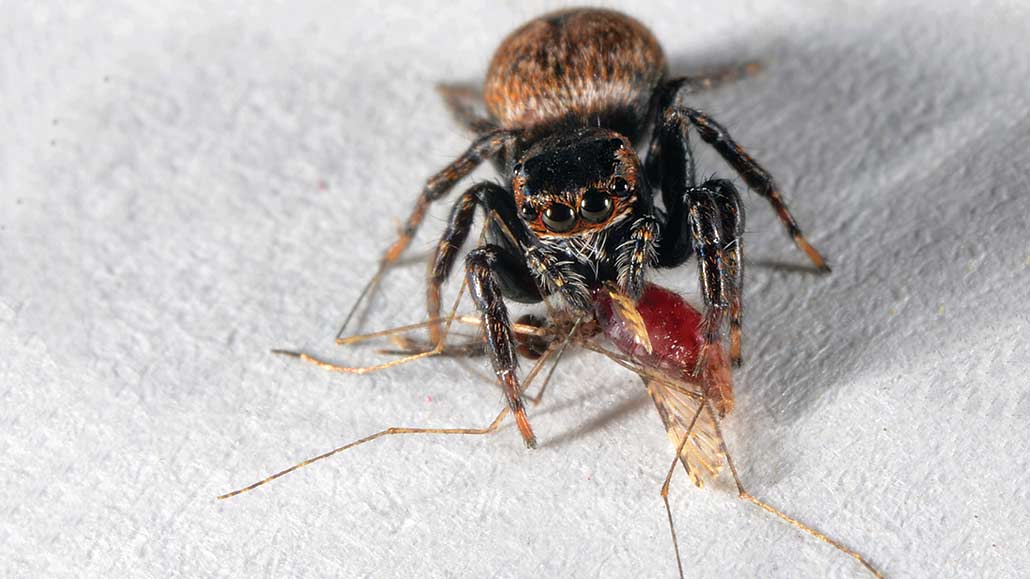The image captures a close-up view of a black and brown, hairy spider situated on a white surface, possibly resembling a paper towel. The spider is centrally positioned in the photograph, directly facing the camera, with its body prominently displayed. Its rounded abdomen is covered in brown hairs, while its eight legs are mostly black adorned with occasional brown specks, tapering off to amber-brown tips. The spider has four visible eyes, two larger ones above its fangs and two smaller ones on the sides of its head.

The spider is in the act of consuming a long, thin insect, which appears to be a mosquito. The insect's translucent tan wings and skinny, tan legs are noticeable against the white backdrop. Red ooze is visible beneath where the mosquito has been killed, adding a stark contrast to the scene. The photograph highlights the intricate details of the spider's anatomy, including its fangs and hairy features, as well as the dramatic moment of its predation.